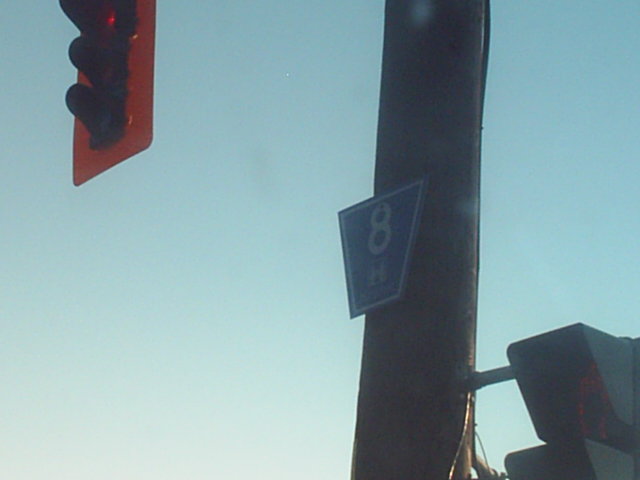This is a landscape-oriented photograph capturing a wooden utility pole with a distinctive blue trapezoid-shaped sign that has the number '8' and an 'H' within a box, all in white text. The pole supports a set of traffic lights, both positioned at the top and center. Both traffic lights are currently showing red, indicating 'stop'. The image also captures another set of signals or possibly crosswalk lights housed in a black square in the bottom right corner. The scene is set against a clear blue sky that gradually fades lighter towards the horizon. In the top left corner, a traffic signal is partially visible, hanging out of frame. The overall day is bright, with no clouds in sight, creating a vivid, yet slightly blurry, mid-day atmosphere.